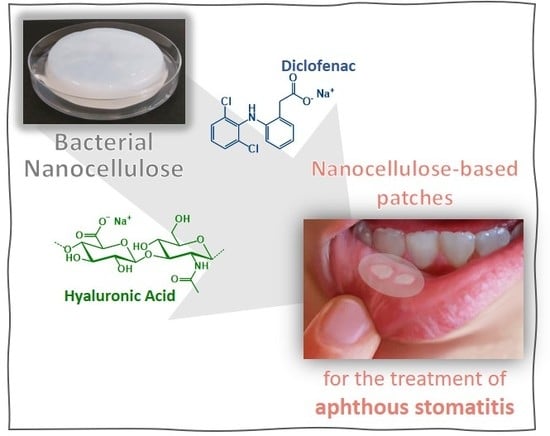The image is a detailed informational poster with a white background and a wavy, thin black border. The poster is divided into four quadrants, each featuring different elements related to a medical topic.

In the top left corner, there's a black square containing a clear circle with a white circle in the center. Below this, the label reads "Bacterial Nanocellulose," and an arrow points downward to the bottom right quadrant.

In the top right quadrant, a structural formula for the organic compound diclofenac is displayed, showing its chemical structure consisting of two full hexagons, a partially completed hexagon in the middle, and a Y-shaped piece to the right. The chemical symbols included are Cl, H, Cl, O, O, and Na, written in blue text.

The bottom left quadrant similarly displays the structural formula for another organic compound, hyaluronic acid. This formula is notably more complex, resembling interconnected bow ties with various lines and Y-shapes extending outward. The chemical symbols are HO, O-, OH, Na+, and NH, among others, written in the formula.

The bottom right quadrant shows an image of a person pulling down their bottom lip with their thumb, revealing a clear disc applied to two white sores inside the lip. The label beneath this image reads, "Nanocellulose-Based Patches for the Treatment of Aftous Stomatitis," with text in red letters. This part of the poster illustrates the application of the medical patch for treating canker or cold sores.

Accompanying the main components are textual labels providing detailed descriptions of each item to clarify the content and purpose of each depicted element.